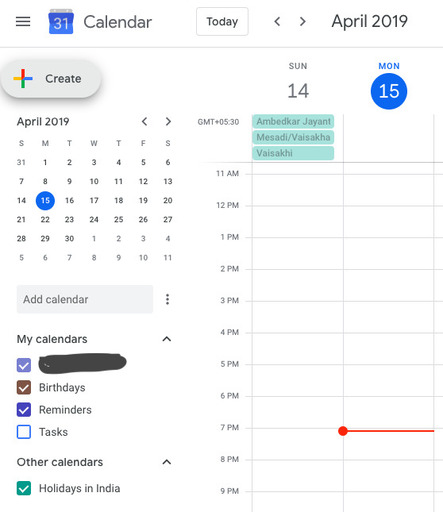This image depicts a digital calendar interface, likely from a website. At the very top, the header reads "Calendar" in black text, accompanied by a "31" in blue, possibly representing a calendar icon. Below the header, there is a navigation bar that includes a "Today" button highlighted with a square around it, left and right arrows for navigating through dates, and the current month and year, "April 2019," displayed prominently.

Directly beneath this navigation bar is a "Create" button in the form of a small oval icon, which features a plus sign in the vibrant colors of Google—red, blue, orange, yellow, and green. Reiterating the current month, "April 2019" is also printed below the "Create" button. A notable detail is that April 15th is marked with a blue circle, indicating a significant date.

Below the calendar grid, there's a gray bar labeled "Add Calendar," followed by the section "My Calendars." Within this section, the first calendar item appears to be crossed out with a black marker. The remaining items, "Birthdays" and "Reminders," have checkboxes next to them, both of which are checked. The "Tasks" item is listed but not checked. Further down, under "Other Calendars," the "Holidays in India" calendar is checked as well.

The right side of the calendar shows a detailed view starting from Sunday, April 14th, to Monday, April 15th—the latter being highlighted with a blue circle around the date. The daily schedule beneath Monday features time slots ranging from 11 a.m. to 9 p.m. Notably, there is a time slot at 7 p.m. that is outlined in red with a small red dot on the left side of the time bar, indicating a scheduled event or reminder for that time.